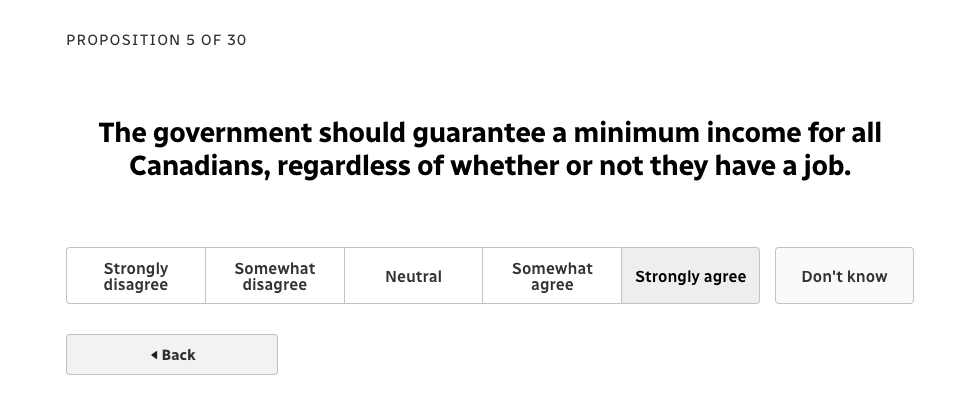This image features a survey interface focused on Proposition 5030, which advocates for the government to guarantee a minimum income for all Canadians, regardless of employment status. The interface presents options for respondents to express their agreement or disagreement with the proposition. The response options include: Strongly Disagree, Somewhat Disagree, Neutral, Somewhat Agree, Strongly Agree, and Don't Know. Additionally, a 'Back' button is available for navigation. The selection marked in this instance is 'Strongly Disagree.' The background of the survey screen is plain white, devoid of any additional imagery or design elements. The text is clearly legible against this minimalistic backdrop.